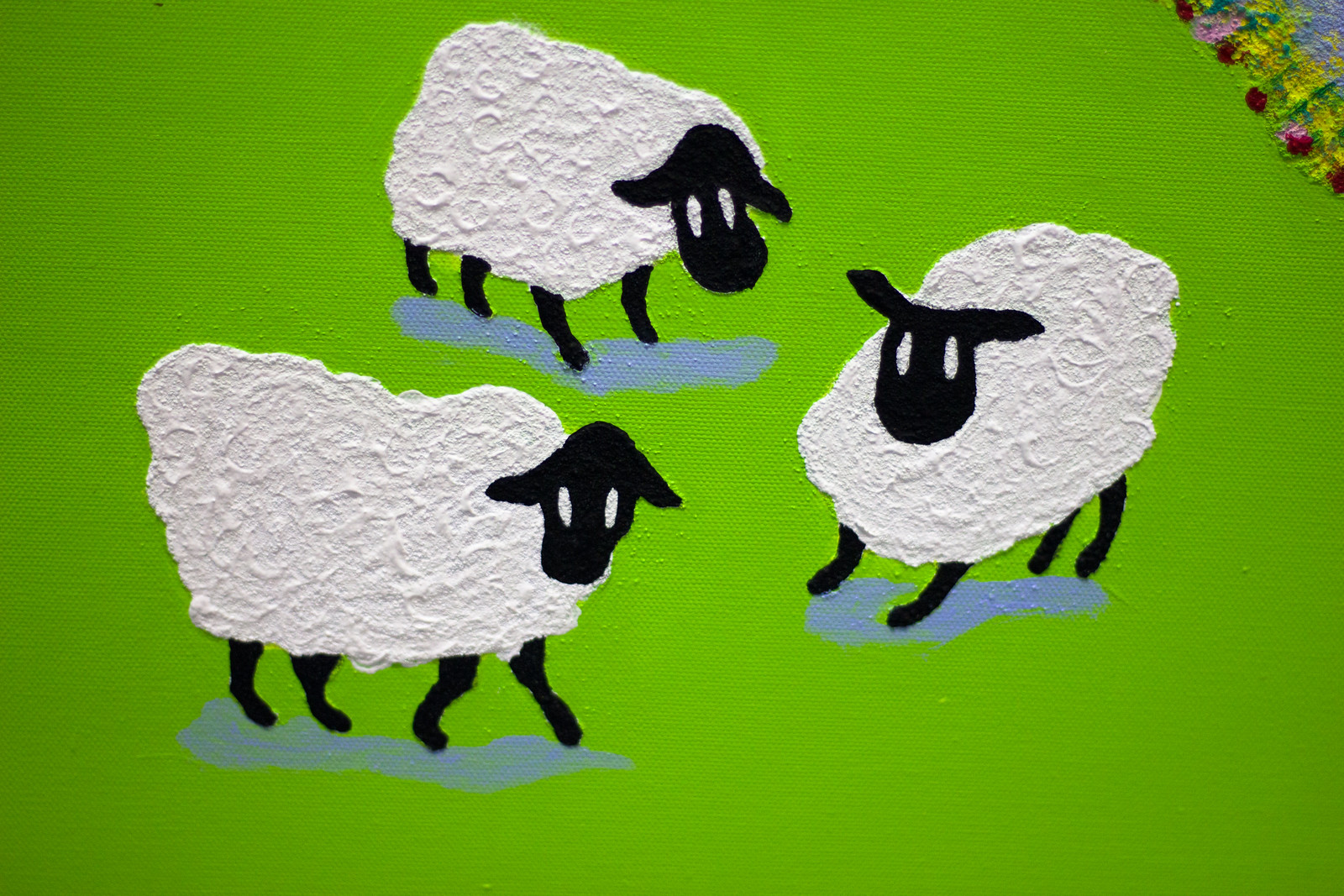The image features a detailed piece of artwork showcasing three sheep. These sheep are depicted with white, textured wool and distinct black heads and legs. Their eyes are oval-shaped and white, adding an expressive touch to their characters. The background is a bright green, possibly acrylic paint, with the foreground sheep casting blue-hued shadows beneath them, which might suggest water or simply artistic choice. Two sheep are prominently positioned at the front while the third stands slightly back. The sheep on the right has a circular face, the left one a square face, and the rear one an oval face with its head facing upward. In the upper right corner of the painting, there's a playful mix of red, yellow, and blue paint splotches, suggesting an experimental touch. The sky above them is very cloudy, enhancing the overall atmosphere of the scene.